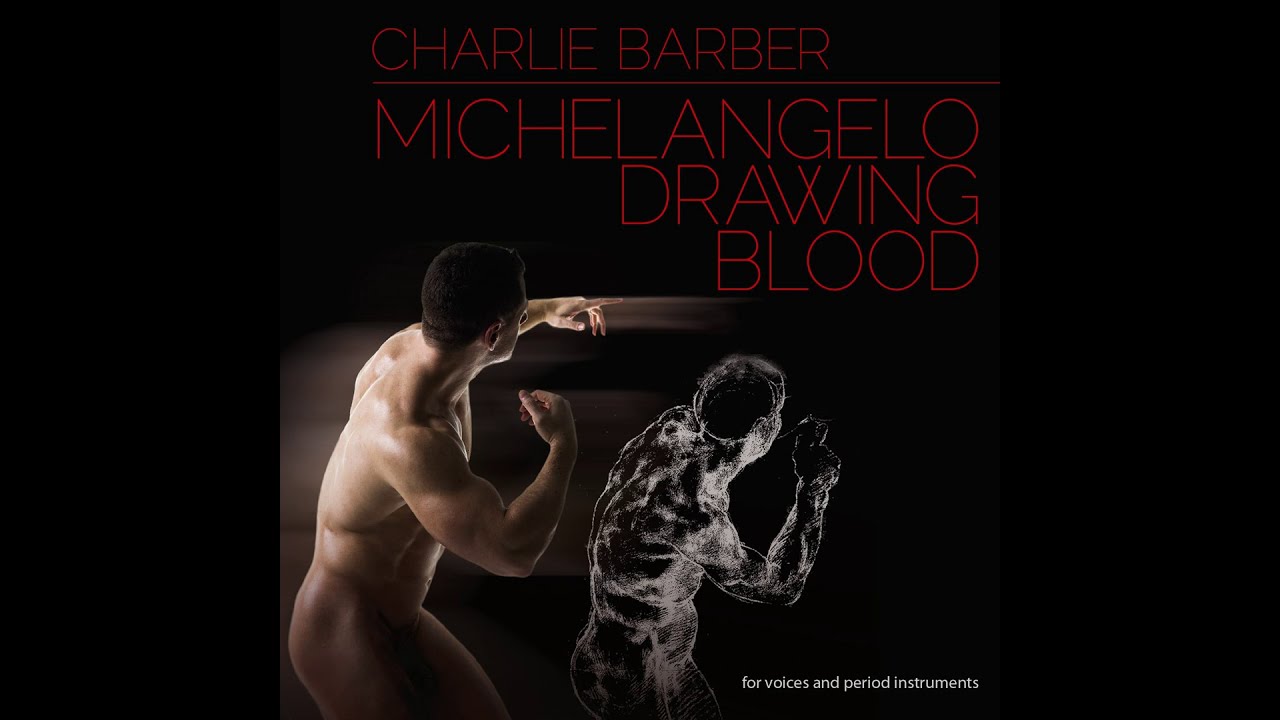The image features a computer-generated design with an all-black background and black borders on the left and right, creating a square format. At the top center, large red letters spell out "Charlie Barber," underlined for emphasis. Directly below that, in even larger bold red capital letters, it reads "MICHELANGELO DRAWING BLOOD." Dominating the center of the image is a nude man with short dark hair, striking a muscular pose reminiscent of a boxer or fighter, with his right arm bent and forming a fist, while his left elbow is raised. Beside him is an artistic sketch replicating the same pose, rendered in white outline, detailing his muscular form. At the bottom right corner, the text "For Voices and Period Instruments" is displayed in white font, adding a classical element to the dynamic scene.